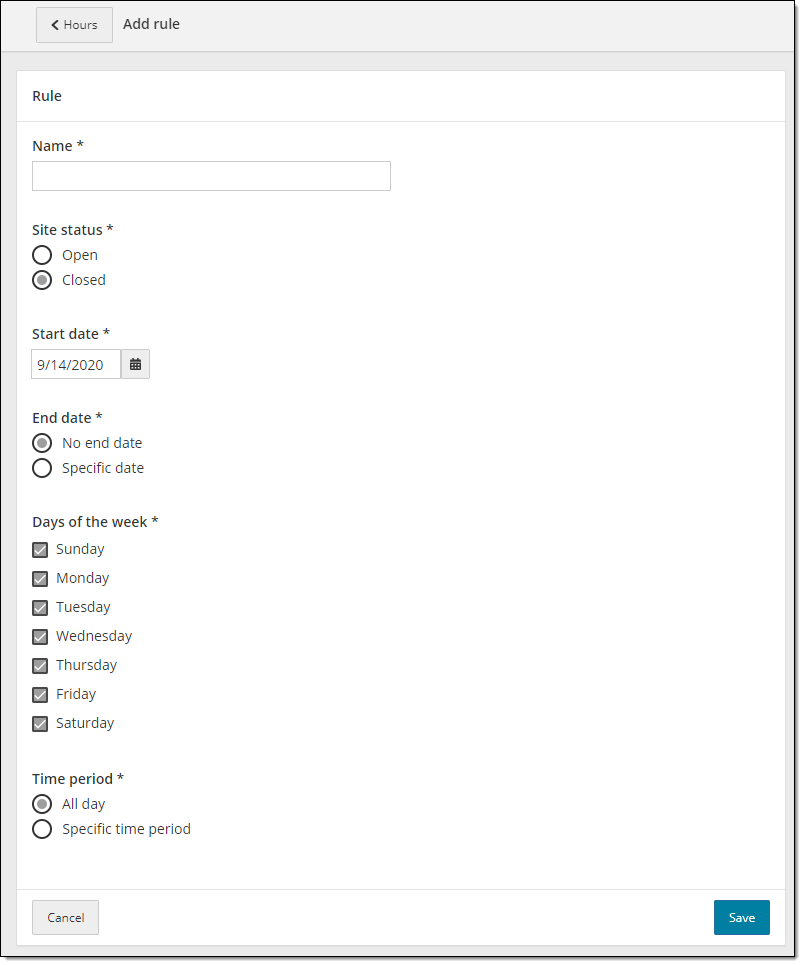This image is a screenshot captured from a section of a webpage, likely viewed on a tablet computer due to its tall and narrow aspect ratio. The overall background of the webpage is white, while the header at the top is gray. The header displays two primary options: "HOURS" on the left and "ADD RULE" on the right.

Beneath the header, the webpage is segmented into various sections labeled "RULE" and "NAME," accompanied by a large input box where the user can type the rule's name. Below this, "SITE STATUS" options are presented with radial buttons allowing the user to select either "open" or "closed." Further down, start and end dates can be specified in designated input fields. 

The days of the week are listed in a column format, each accompanied by a small checkbox. In this screenshot, all seven checkboxes for the days of the week are marked as checked. At the bottom of the form, "TIME PERIOD" options are available, with choices for "all day" or "specific time period." In this instance, "all day" is selected.

In the lower right-hand corner of the webpage, there is a blue rectangular button labeled "SAVE" in white text, ready to be clicked to confirm the inputted settings.